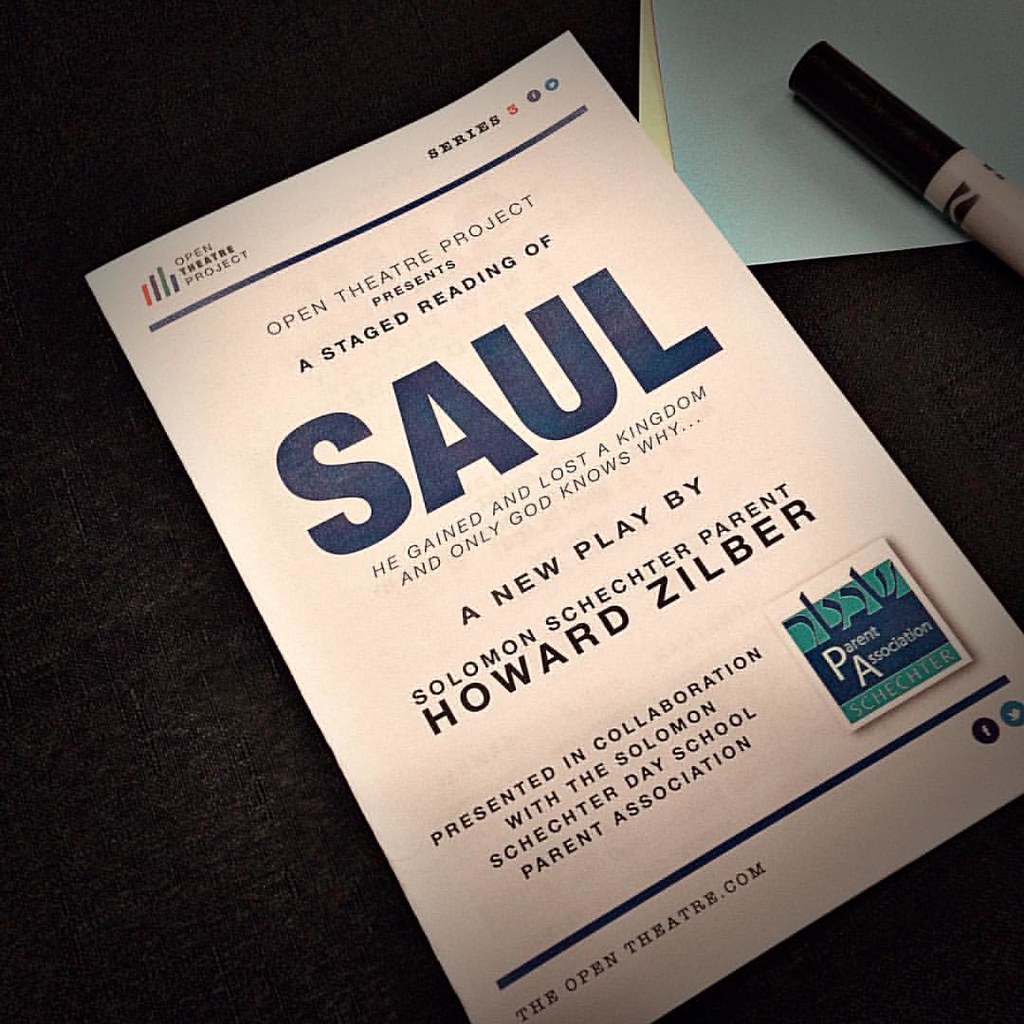This is a detailed photograph of a playbill positioned diagonally on a dark gray or black background. The playbill is from the Open Theater Project's Series 3, featuring a staged reading of a new play titled "Saul." At the top left, the text "Open Theater Project" is displayed alongside their logo, consisting of four slanted vertical lines in different colors. A blue horizontal line separates the header from the main text below. The main title "Saul" is prominently written in large, blue, all-capital letters, followed by the subheading, "He gained and lost a kingdom and only God knows why."

The play is attributed to Solomon Schechter parent, Howard Zilber. The information continues with the note that the presentation is in collaboration with the Solomon Schechter Day School Parent Association, whose logo appears on the right side of the playbill in both dark blue and light green. At the bottom, after another blue horizontal line, the left side reads "TheOpenTheater.com" while the right side contains Facebook and Twitter logos, the former in dark blue and the latter in light blue.

Additionally, in the upper right corner of the photograph, there is a piece of yellow paper with a smaller piece of light blue paper on top, and a black magic marker resting on it.